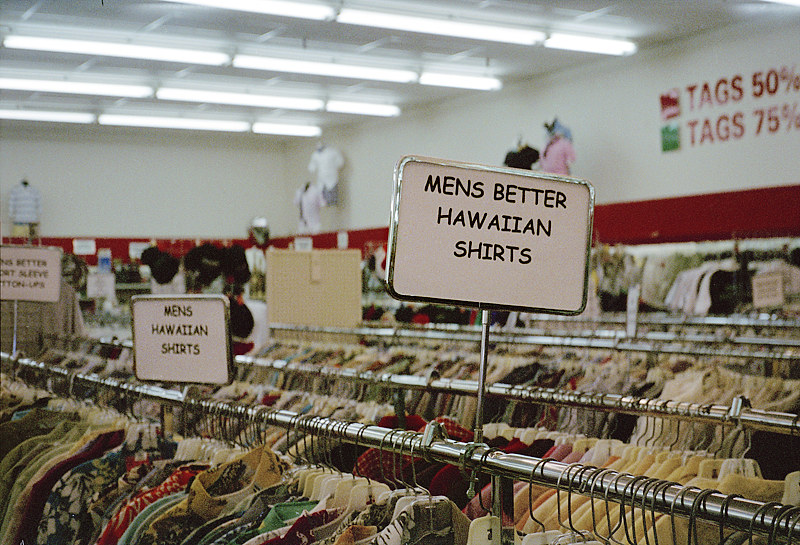The image captures the vibrant interior of a discount department store, specifically highlighting a section dedicated to men's Hawaiian shirts. Prominent signs announce significant discounts, with red tags indicating 50% off and green tags signifying 75% off, as explained by a sign on the wall located in the upper right-hand corner of the photo. In the foreground, a sign prominently reads "Men's Better Hawaiian Shirts," while directly behind it, another sign labels a rack as "Men's Hawaiian Shirts." Further back, although partially obscured, a third sign appears to read "Better Short Sleeve Button-Ups." This section is filled with numerous racks teeming with colorful Hawaiian shirts, creating a lively and tropical atmosphere within the store.